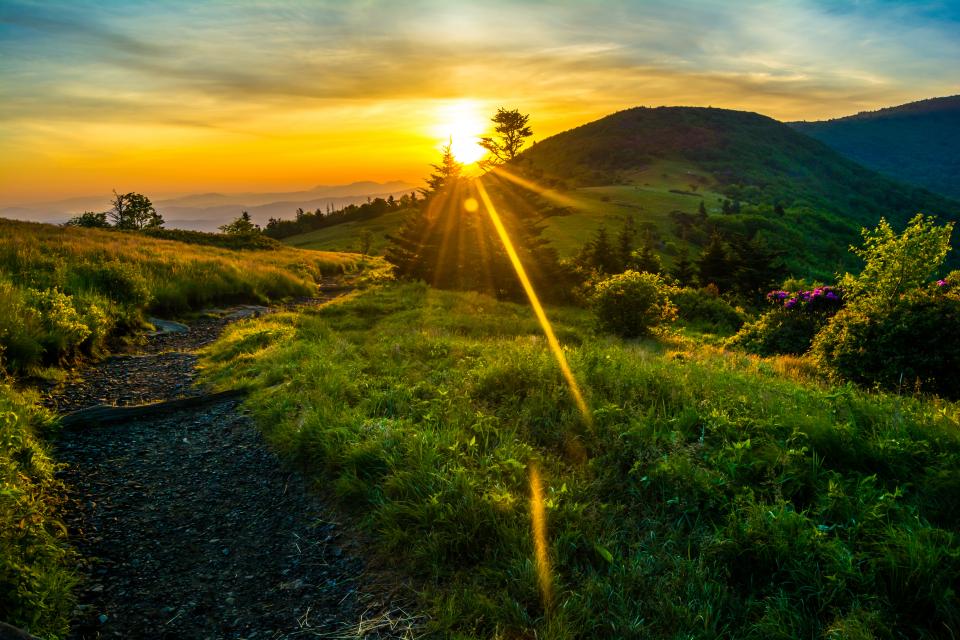A rectangular landscape photograph, with the longer side extending horizontally, vividly captures a serene nature scene. The vantage point appears to be from one hill, offering a captivating view of an adjacent hill during what seems to be either a majestic sunrise or tranquil sunset. The foreground features a well-maintained trail, lined with rocks and pebbles, meandering from the bottom edge and curving towards the center. On each side of the trail lies a lush grassy expanse, interspersed with bushes. Among these bushes on the right side, hints of purple flowers peek through the greenery. 

Dead center in the background, a clump of sizable trees stands prominently, while a solitary tree is visible further in the distance, precisely at the point where the radiant sun begins its ascent or descent. The sun itself casts a brilliant glow, transitioning from a bright yellow-white core to golden hues that gradually blend into the surrounding sky. To the upper right, a large grassy hill rises, with additional rolling hills fading into the distance. The sky above is a blend of haze and clouds, with a touch of blue faintly visible at its zenith, completing this picturesque natural tableau.